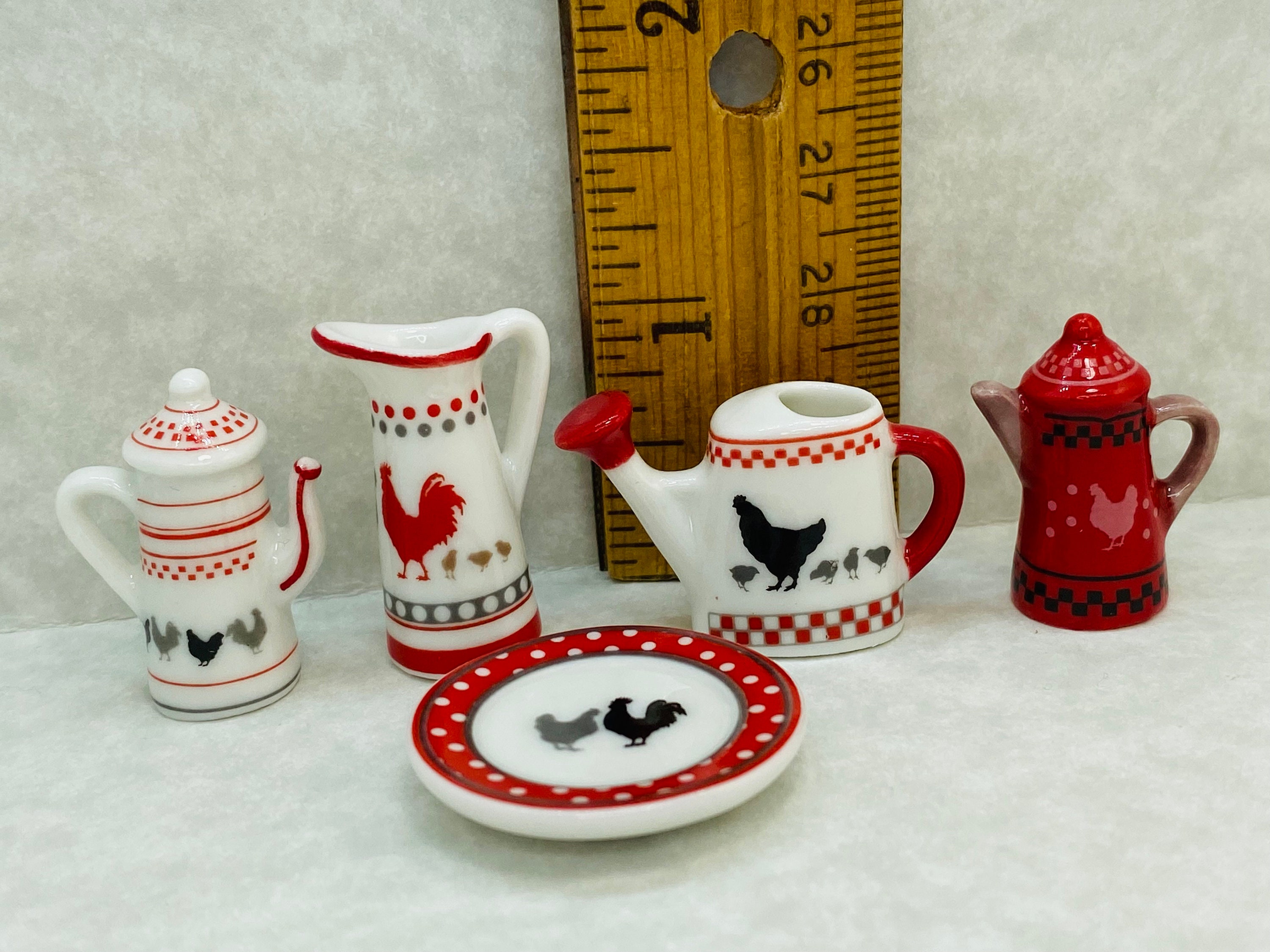This photograph showcases a charming, miniature farmhouse tea set displayed against a white background with a wooden ruler in the backdrop, indicating the set pieces are each approximately one inch tall. The set includes five pieces: one white plate and four pitchers, each adorned with detailed rooster and chicken illustrations. The plate features a red rim adorned with white polka dots and showcases a central design of a black chicken and rooster. Among the pitchers, one stands out with a red color and intricate black patterns near the top and bottom edges, displaying a white chicken. Another is white with a red handle and spout, decorated with red checkered patterns and a prominent red rooster front and center. The third pitcher, resembling a water can, has a red tip and handle, red and white checkered bands at the top and bottom, and a black chicken followed by four smaller chicks. Emphasizing the farmhouse theme, the tea set combines white and red hues with charming poultry motifs, creating an adorable and detailed miniature playset.